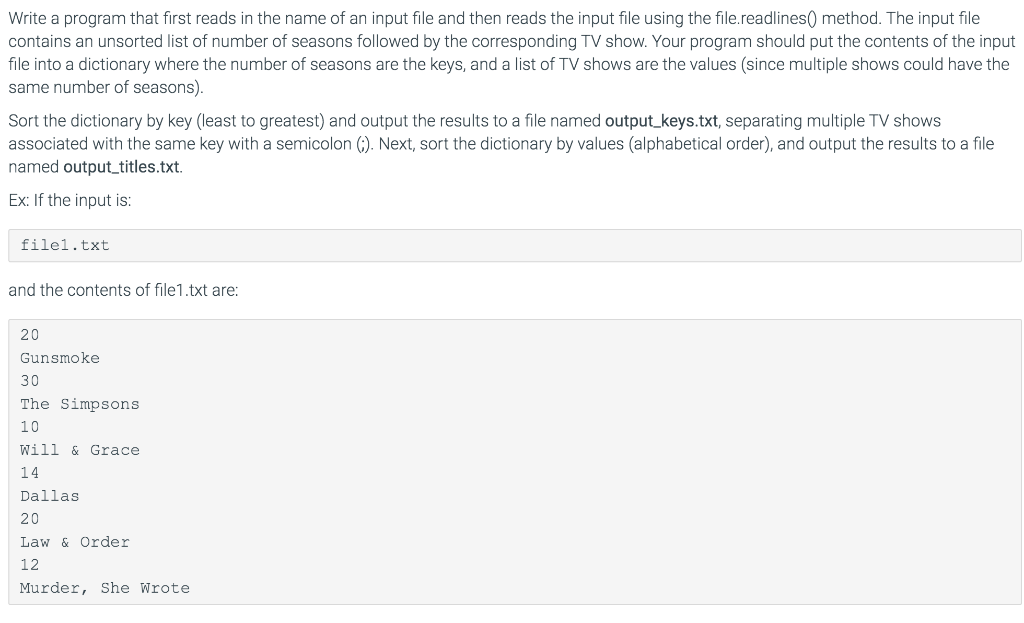**Descriptive Caption:**

The image contains a block of black text on a plain white background. The text outlines a programming task that requires writing a program to process an input file. This input file contains an unsorted list of the number of seasons followed by their corresponding TV show. The program should employ the `readlines` method to read the file and then store the contents in a dictionary, where the number of seasons serve as keys and the associated TV shows are stored as values in lists. In cases where multiple TV shows share the same number of seasons, they should all be listed under the same key. 

The program is required to sort this dictionary first by the number of seasons (least to greatest) and output the results to a file named "output-titles.txt", with multiple TV shows for the same season count separated by a semicolon. Following this, the program should sort the dictionary by the TV show names in alphabetical order and save the results to the same output file.

For instance, given an input file "file1.txt" with the following content: 

```
20, Gunsmoke
30, The Simpsons
10, Will & Grace
14, Dallas
20, Law & Order
12, Murder, She Wrote
```

The program should handle this data as per the specified instructions. The task description abruptly ends, leaving the conclusion unknown.